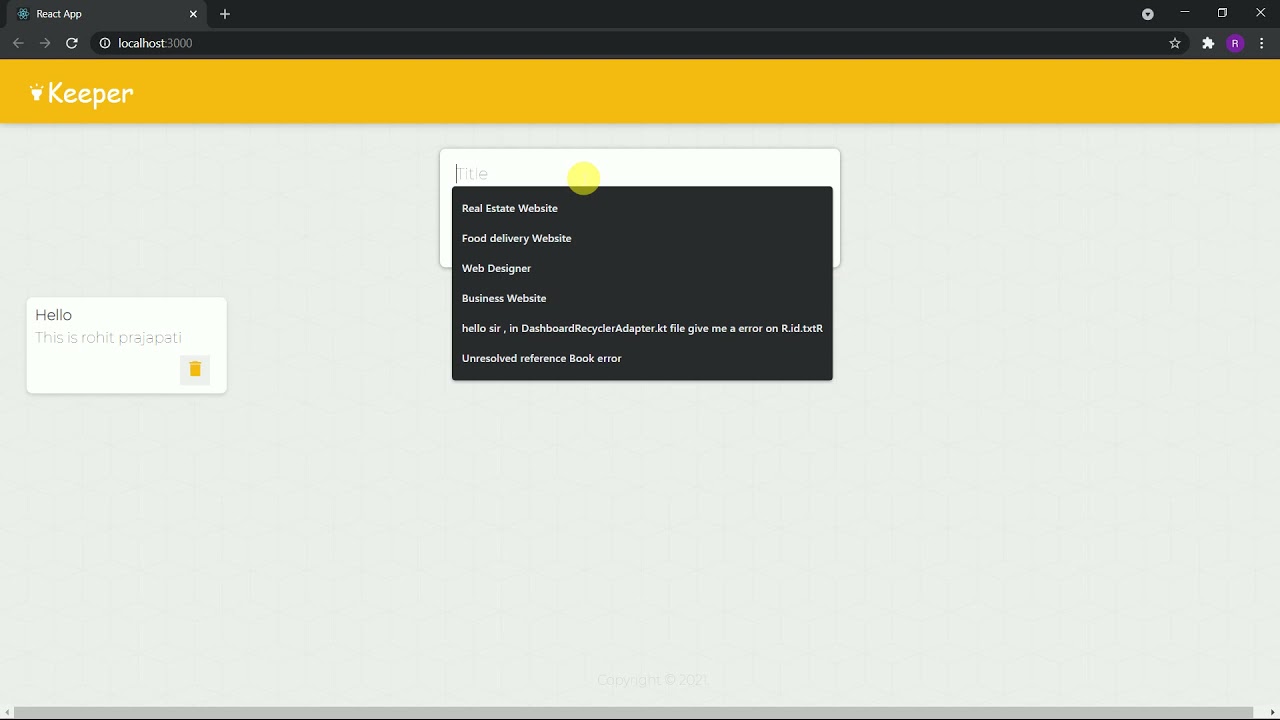Screenshot of a website in dark mode, indicated by the dark gray browser bar at the top and the address "localhost:3000" in the white address bar. The website features a mustard yellow header with the word "Keeper" in the top left corner, accompanied by a white downward-facing caret to the left of the word. The main background of the website is gray.

In the left center of the screen, there is a prominent white rectangular text box displaying the message "Hello" in black text, followed by "This is Rohit Prajadati" in gray text underneath. An orange trash can icon is located in the bottom right corner of this white text box, presumably for deleting the message.

At the center top of the screenshot, there is a user text entry box, which has been selected, revealing a gray drop-down menu with suggested titles for user input.